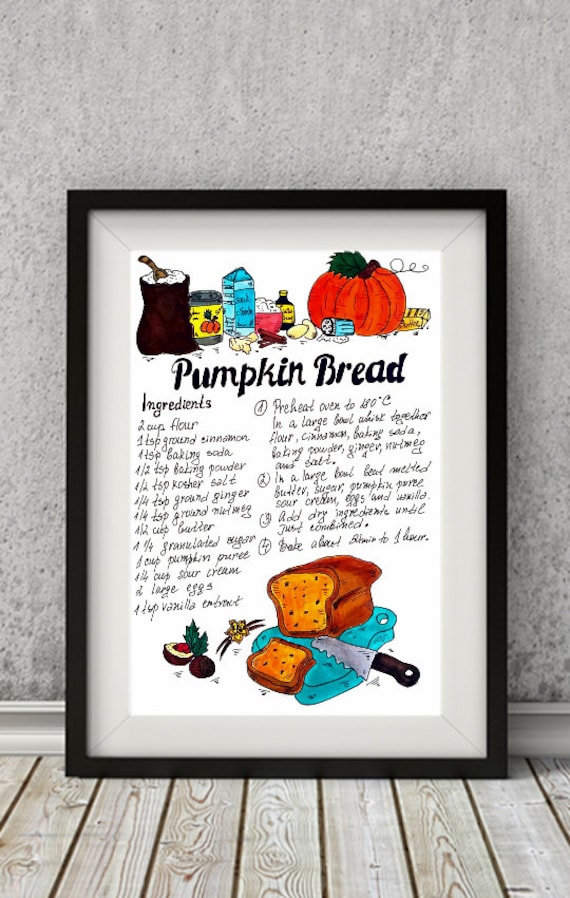This image showcases a framed recipe for pumpkin bread, leaning against a gray textured wall on a wooden floor. The black-framed piece features a white background with black text detailing the pumpkin bread recipe, including essential ingredients such as 2 cups of flour, 1 teaspoon each of ground cinnamon, baking soda, baking powder, and kosher salt, and 1 1⁄4 teaspoon of ground ginger. The recipe and instructions are slightly difficult to read due to the small text. Above the title "Pumpkin Bread," colorful drawings depict various ingredients like a pumpkin, eggs, butter, vanilla extract, and a blue milk carton, adding a charming, country-art style to the piece. The bottom of the recipe includes a vivid illustration of an orange and brown loaf of pumpkin bread on a blue cutting board, with one sliced piece, a knife, and some decorative elements like herbs and possibly a halved avocado.